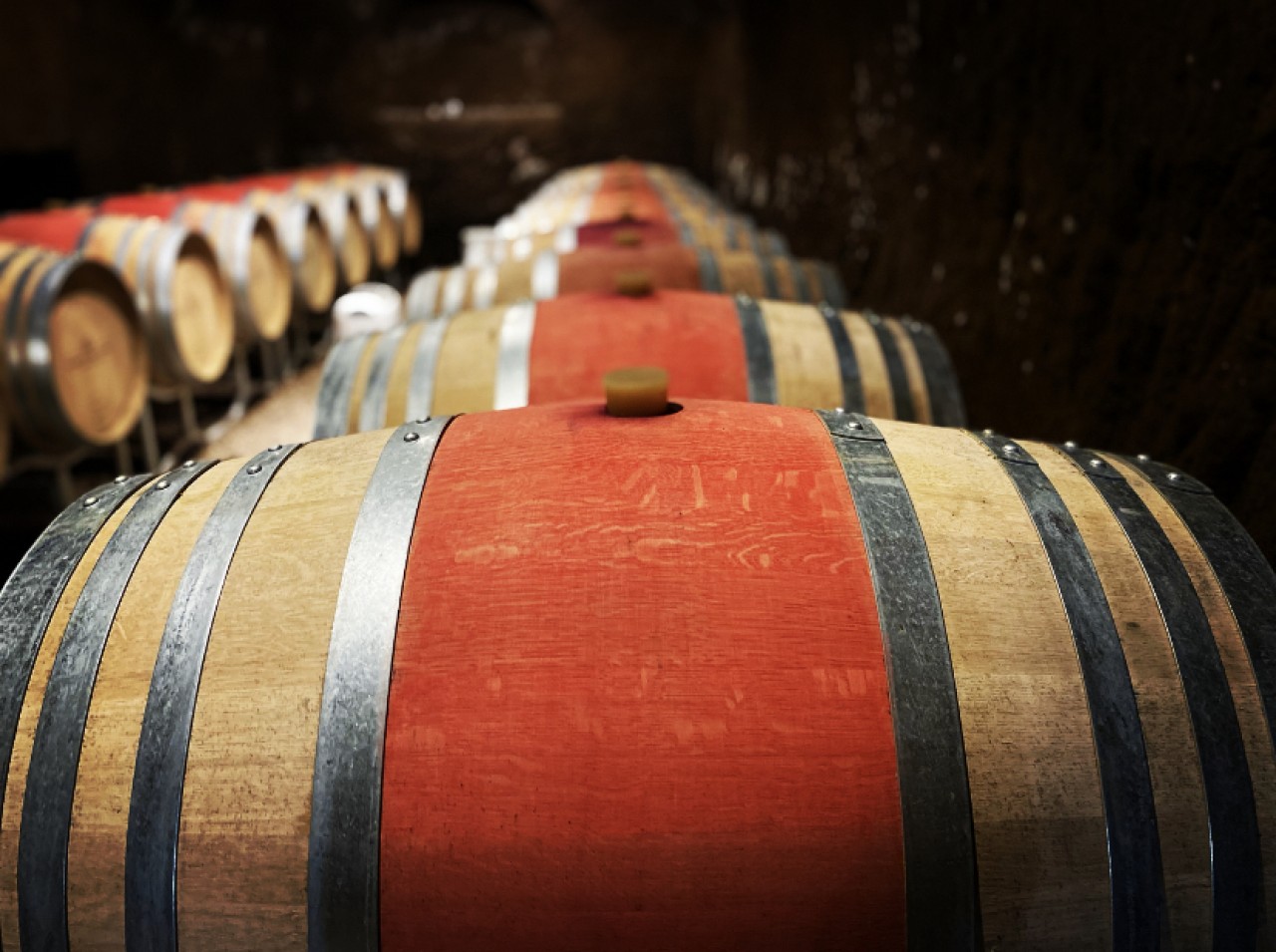This detailed color photograph captures two rows of wooden barrels, likely oak, lying horizontally in a cellar-like environment. Each barrel features a center section painted a vibrant reddish-orange, flanked by sections of natural light-colored wood. Every barrel is secured with multiple metal bands, specifically two around the painted section and three on each side of the natural wood, totaling eight metal straps per barrel. Visible corks or openings are found at the top center of each barrel, presumably used for testing, filling, and refilling the contents. The barrels rest on what appear to be small metal stands, preventing them from rolling. The illumination from an external light source or camera flash highlights the barrels against the darker, cavernous room, with one row of barrels in sharp focus and the second, parallel row slightly blurred, creating depth in the photograph. The composition suggests a storage area extending, with approximately 15 to 20 barrels in the visible row.